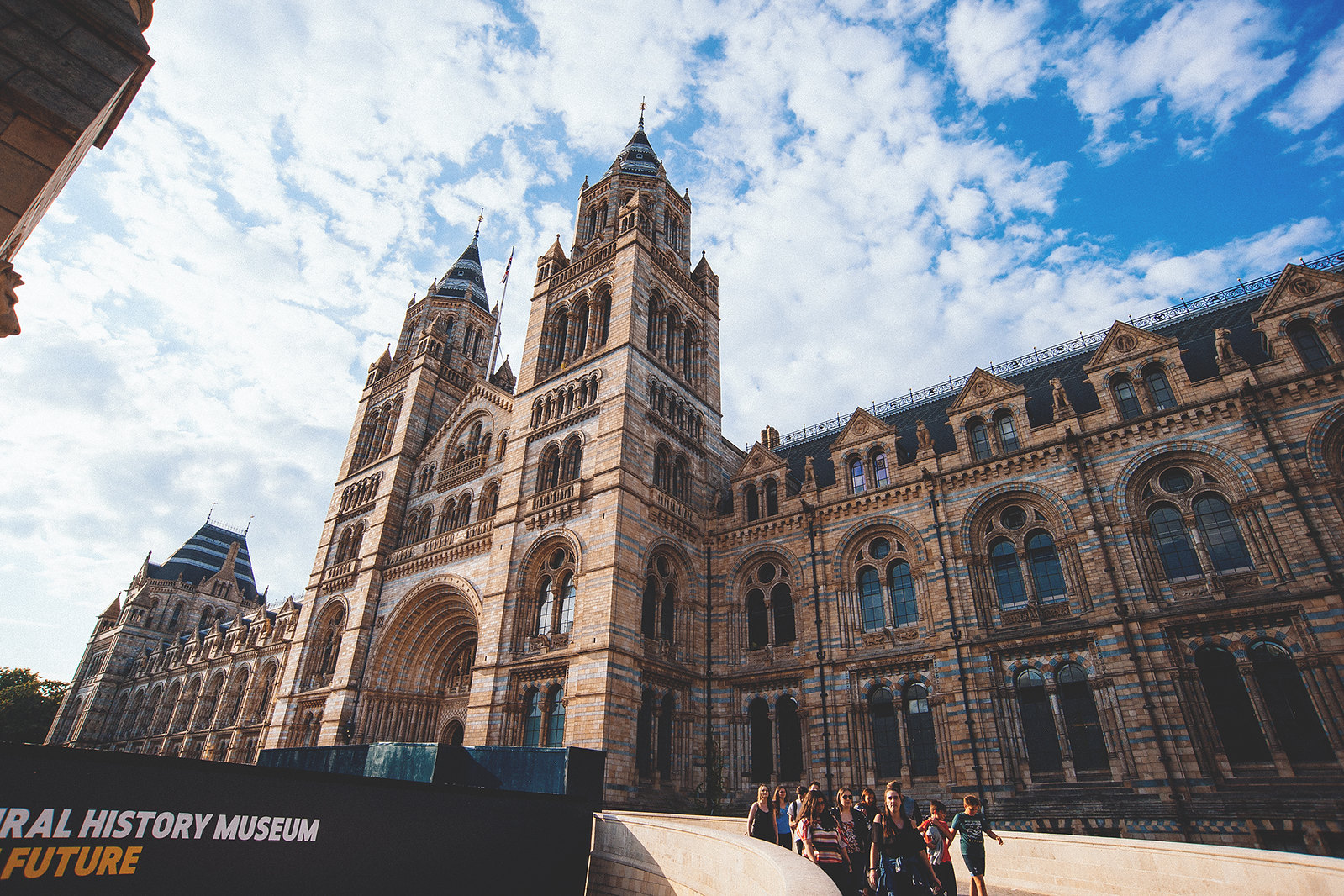A large, stately building resembling a cathedral dominates this outdoor image taken on a cloudy day. The structure, made of tannish-red brick with grey accents, features an impressive facade with arched Gothic windows, numerous steeples, and two five-story towers flanking the main arched entrance. The building is labeled as a museum, with a partially visible sign reading "History Museum Future" in the bottom left corner. In the upper left corner, part of another building is visible. The scene is bustling with people, likely visitors, congregating and walking on a path before the grand edifice. The sky overhead is mostly cloudy with some patches of blue. A woman wearing a black t-shirt stands at the forefront of the group in the right bottom corner.